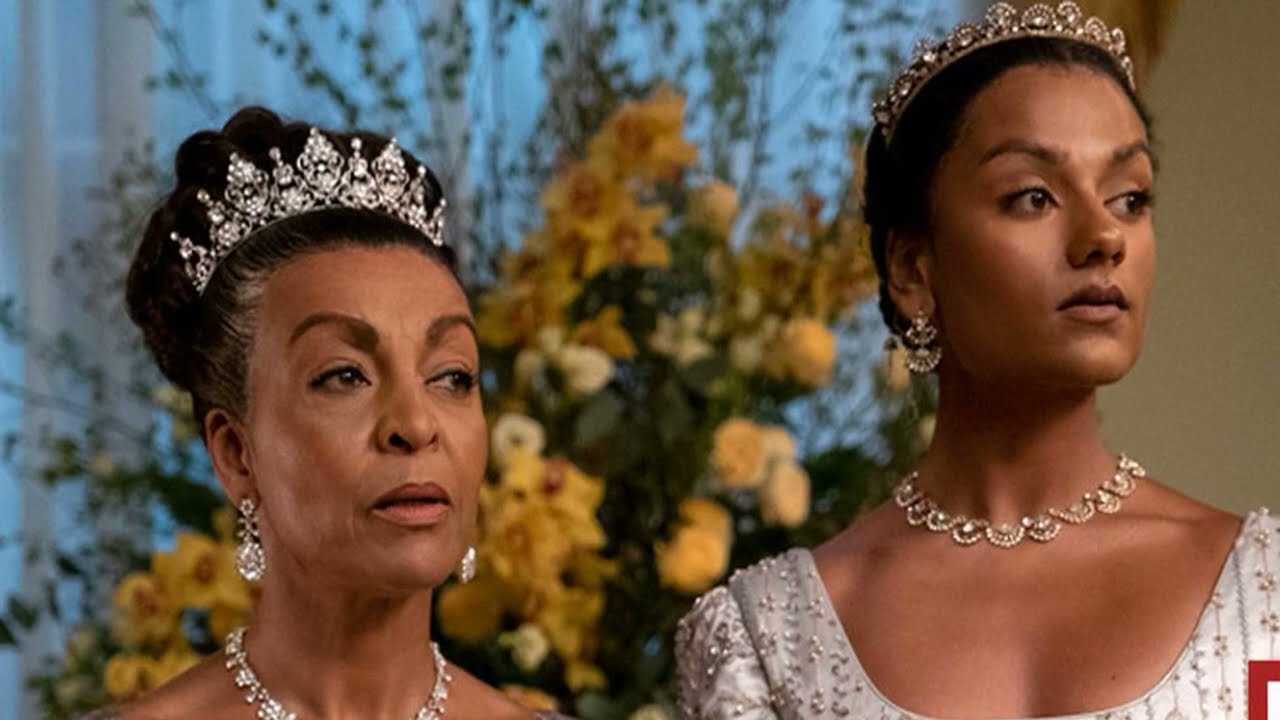The image appears to be a screenshot from a video or movie scene, resembling something like "Bridgerton." It depicts two dark-skinned women who appear to be of royal status, wearing elaborate jeweled tiaras and diamond-studded necklaces. The woman on the left is older, possibly in her 50s, with her hair swept back and adorned with large teardrop-shaped diamond earrings. She wears a fairly ornate and large tiara. The younger woman on the right, possibly in her 20s, sports a less high but intricately designed tiara and scallop-shaped diamond enclosures around her neck. Both women are gazing slightly to their left. In the background, a blurry, large assortment of flowers and a blue curtain or cloth can be seen. The image captures them from their chests up, highlighting their regal and detailed attire.